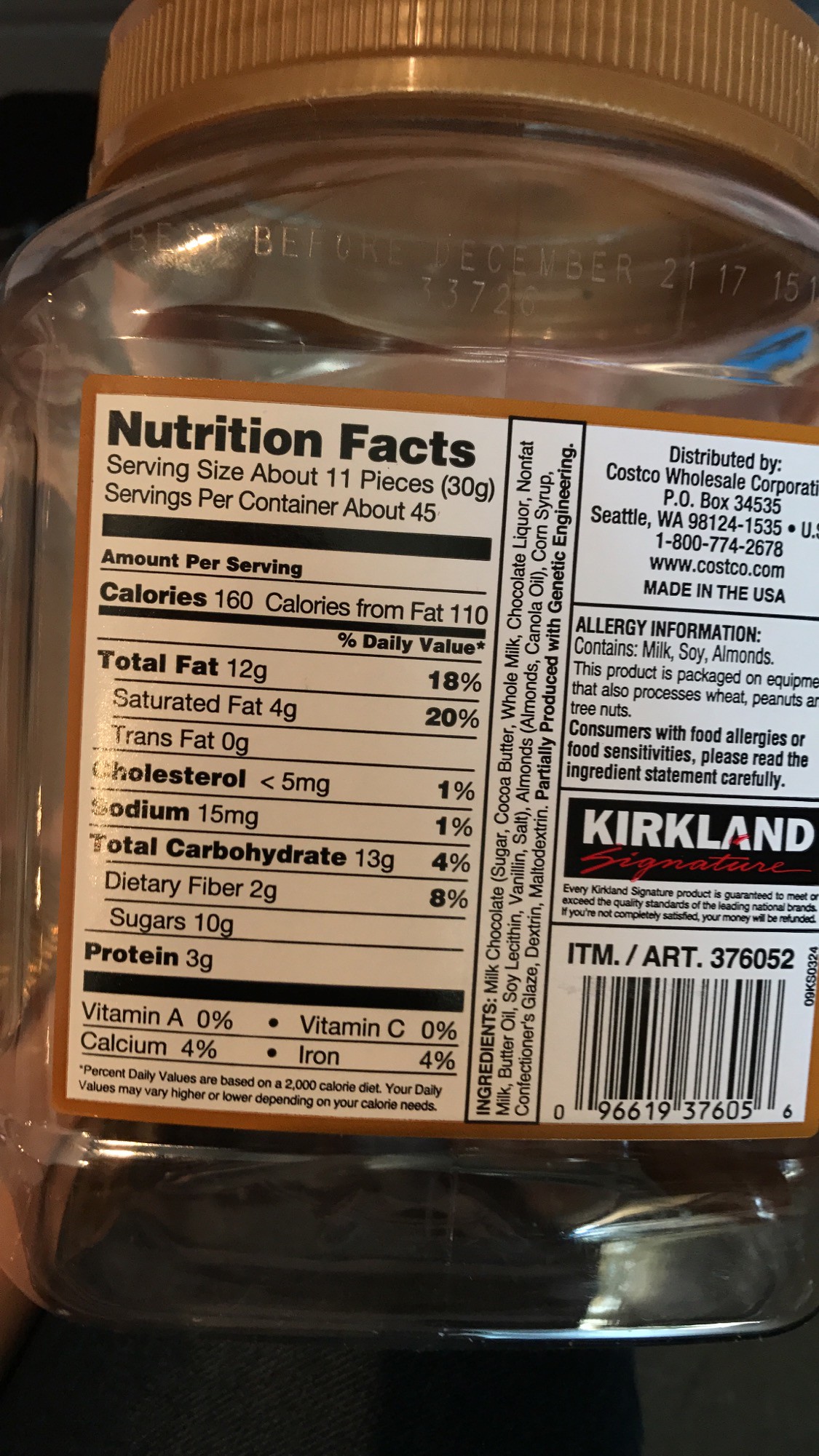The image showcases the back of an empty, clear plastic jar that typically holds nuts. The jar, comparable in size to standard peanut containers, features a brown screw-top lid. Prominently displayed is the nutrition facts panel, which indicates that a serving size is approximately 11 pieces, with a total of 45 servings per container. Each serving contains 160 calories, 110 of which are from fat. The detailed nutrition information adheres to standard labeling formats.

This empty container was distributed by Costco Wholesale, under their Kirkland brand. It contains allergy warnings for milk, soy, and almonds, suggesting that the jar originally held a nut-based product, perhaps almonds. A barcode can be found at the bottom right of the label. The jar, now devoid of its contents, hints at its previous role in storing nutritious snacks.